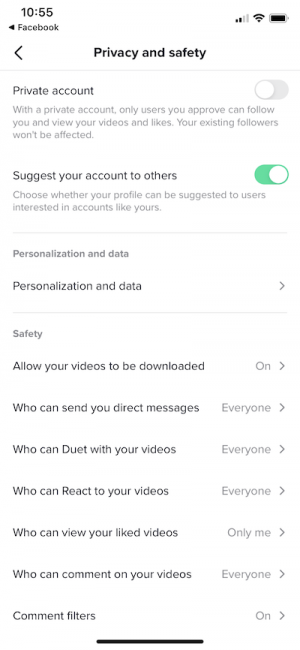The image is a screenshot of a smartphone displaying the "Privacy and Safety" settings of a social media app, likely TikTok. The interface is housed within a thin vertical rectangle, typical of a smartphone screen. 

At the top of the screen, there's a back arrow in the top left corner. Directly below is a heading that reads "Privacy and Safety." Under this heading, the first option listed is "Private Account," which is accompanied by an explanation and an on/off toggle switch set to "Off."

The next section is "Suggest Your Account to Others," which allows users to choose whether their profile can be suggested to other users. This option is toggled to "On."

Following that is the "Personalization and Data" menu that includes various settings, each with options that can be toggled to "Everyone," "Only Me," or "Friends." 

Under "Safety," several settings are listed:
- "Allow Your Videos to Be Downloaded" is set to "On."
- "Who Can Send You Direct Messages?" is set to "Everyone."
- "Who Can Duet with Your Videos?" is set to "Everyone."
- "Who Can React to Your Videos?" is set to "Everyone."
- "Who Can View Your Liked Videos?" is set to "Only Me."
- "Who Can Comment on Your Videos?" is set to "Everyone."

Additionally, there is an option for "Comment Filters," which is turned "On."

The entire screenshot captures the organized structure of privacy and safety settings within the app.